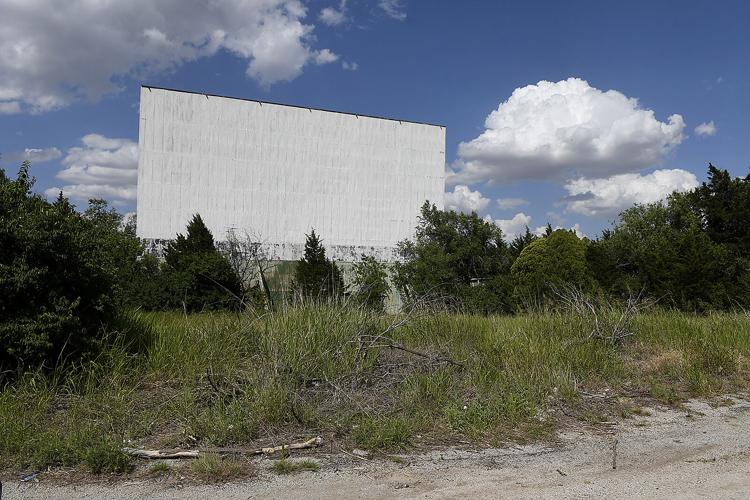The photograph captures an outdoor scene featuring a partially visible dirt road at the bottom edge, characterized by its light beige, sandy texture. In front of the road lies an overgrown field of tall, untamed grass, interwoven with yellowing patches and scattered dead branches. The terrain slightly inclines upwards, giving way to a backdrop of modestly sized trees, some of which are evergreen while the rest exhibit varying shades of green. Dominating the middle background is a large, rectangular billboard that stretches horizontally from the left side of the image towards the center. The billboard is completely blank and stark white, suggesting it was once used for advertisements but is currently empty, possibly awaiting new content. Above this scene, the sky is a vibrant blue, dotted with large, fluffy white clouds that appear to be fairly low. The overall atmosphere suggests a bright, sunny day.